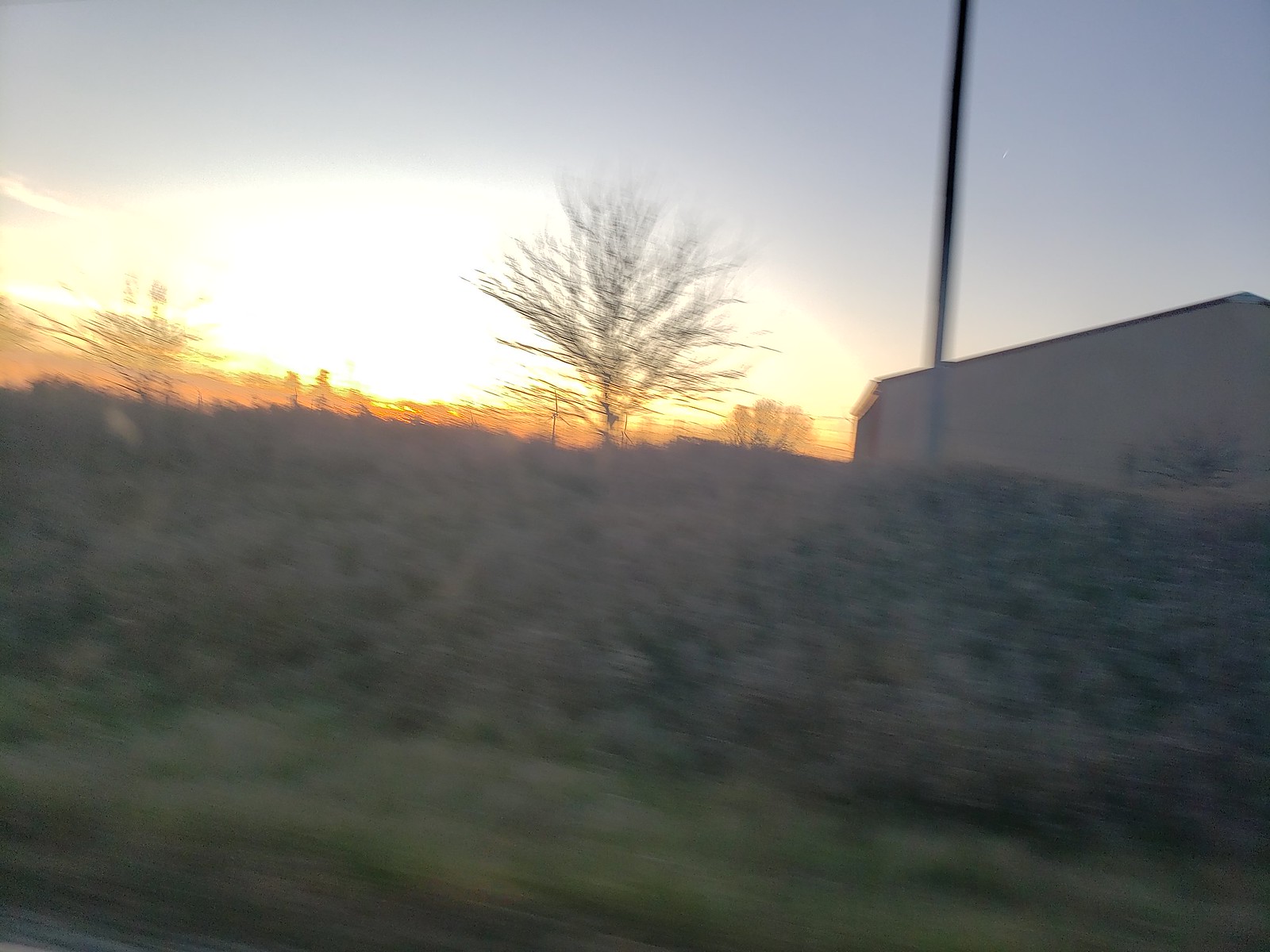The photograph captures a blurred, outdoor landscape scene likely taken from a moving vehicle. The foreground features a slightly rounded mound or raised roadside area, spanning from the left side to the right, angled downwards at about 10 degrees. This section is characterized by indistinct vegetation, with hues of soft greens, grays, and browns, and possibly some gravel and grass. The foreground's indistinct details make it challenging to discern specific elements, though some dead sticks or bushes may be present.

Central to the image stands a prominent, leafless deciduous tree, indicating a winter setting. A slightly smaller tree can be seen in the background. To the right of this main tree is a vertical telephone pole that ascends in front of a large, brown or white warehouse-like building, which extends to the image's right edge. The building is seen from the side, presenting a flat end rather than the roof's slope.

The sky above features a striking, partially visible sun, likely setting or rising, casting a bright, large yellow glow that transitions into an orange horizon line, dominating the left side of the image. The upper sky shifts to a medium gray, creating a vivid contrast against the bright foreground and horizon. The blurred quality of the image and vibrant colors suggest some movement at the time of capture.